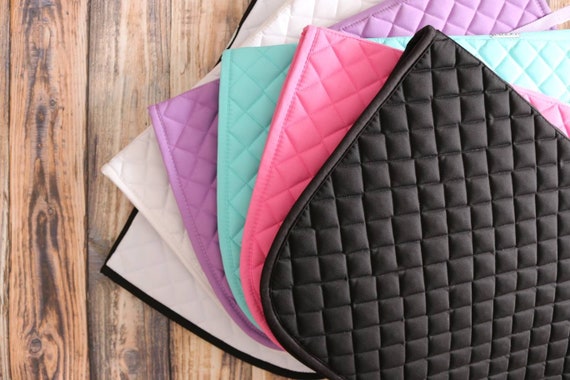The photograph captures several colorful padded mats arranged in a fan-shaped layout on a wooden tabletop. The mats, each designed with a quilted pattern of cushioned squares, extend diagonally across their surface, giving them a plush, pillow-like texture. The mats are layered from top to bottom in this ascending order: black, pink, teal, purple, white, and a final white one with a distinctive black border trim. While most of the mats appear uniform in design, the bottom one seems slightly thinner or made differently, indicating subtle variation. The wooden table, made of vertically aligned planks with a light brown and dark accent grain, provides a contrasting backdrop that enhances the vibrant colors and texture of the mats.